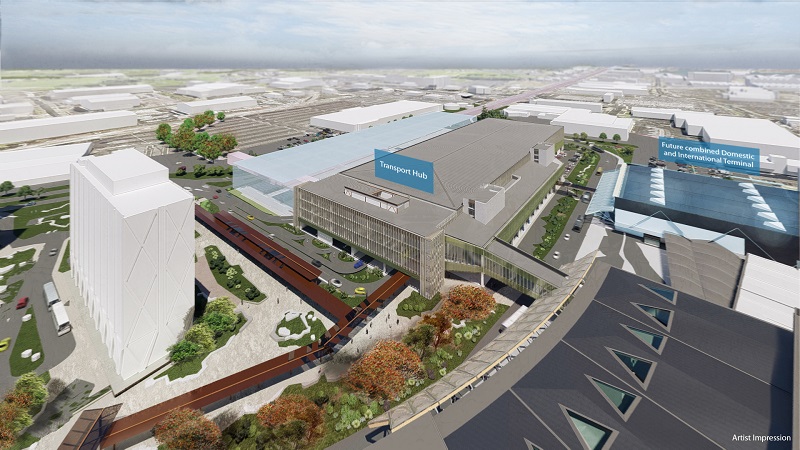This AI-generated image depicts a proposed airport design, viewed from an elevated perspective. Dominating the center is a modern, gray building labeled "Transport Hub" with a prominent blue billboard featuring white text. This structure is surrounded by a variety of other buildings, including a forthcoming "Future Combined Domestic and International Terminal" indicated by a distinct blue and white sign. The setting includes a cloudy sky, giving a muted daylight ambiance. The left side of the image showcases a tall, white, nondescript building accompanied by a parking lot. To the right, there's a covered interior tunnel connecting the main hub to another structure adorned with triangular windows. Several new-looking white flat buildings, possibly aircraft hangars, form the background. The scene includes various vehicles, such as large white buses, a yellow bus, and a small yellow electric car, set amidst realistic-looking trees and bushes that enhance the overall composition.